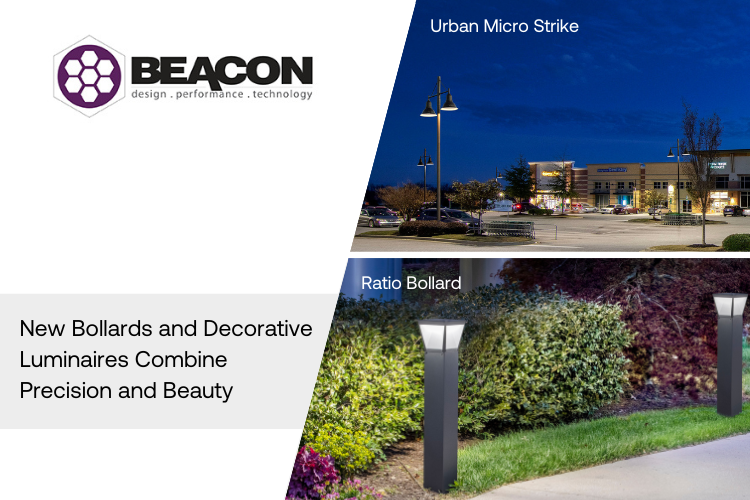The advertisement for Beacon prominently features their honeycomb logo, characterized by a large hexagon housing a black circle with seven nested white hexagons inside. The text states, "Beacon: Design, Performance, Technology." Below this, it proclaims, "New Bollards and Decorative Luminaries Combine Precision and Beauty." 

To the right of this text are two stacked images bisected by a slashed angular line on their left sides, while the outer edges remain straight and 90 degrees. The top image, labeled "Urban MicroStrike," captures an early evening scene at a shopping center or mall, showcasing overhead lights illuminating a parking lot dotted with cars and shopping cart return trays. The bottom image, labeled "Ratio Bollard," is a close-up of two angled gray light fixtures on rectangular posts. These fixtures, with white faces and gray caps, are positioned along a walking path near concrete and grass, backed by neatly trimmed, multi-colored hedges.